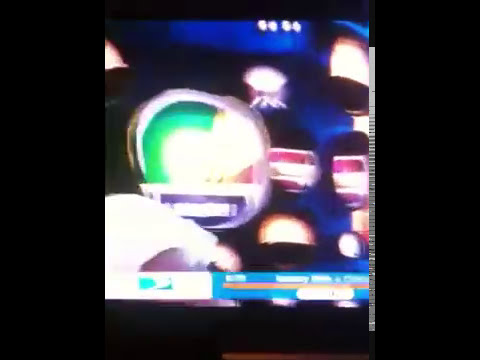The image appears to be a highly blurry photograph of a television screen, characterized by significant letterboxing—approximately 20% on each side and 5-15% from the top and bottom—resulting in a disproportionately reduced central viewing area. The central portion is notably out of focus, making it difficult to discern specific details. The background of the image predominantly features dark blue and black hues. Prominently, towards the bottom left, there is a logo that resembles the DirecTV logo, set within a blue and white strip that spans across the bottom. Along this strip, there is illegible white text and an orange line. In the center-left of the image, there is a circular gauge-like object outlined in green, yellow, and red. Adjacent to this, towards the right, are two smaller circular shapes in red and white. Additionally, a bright oblong circle can be seen a few inches down from the top. The overall impression is of a chaotic, indiscernible scene, possibly from a video game or television broadcast, cluttered with various unidentifiable circular and linear elements.